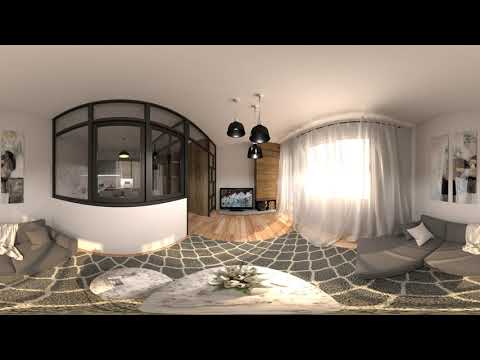The living room, captured in a panoramic view, features walls painted in a light white color, creating a bright and open atmosphere. Dominating the center of the image is a large-screen TV placed on the ground. Above it, three matching black ceiling lamps hang, illuminating the room. 

In the lower center, two tables, one white and one grey, serve as focal points, potentially adorned with flowers. The floor is covered with a grey rug that ties the room together. 

On the right side, there's a grey couch with white cushions and a white throw draped over it, adding a touch of comfort next to a window covered with white curtains, partially allowing sunlight to filter through. Above the couch, various paintings decorate the wall.

To the left, the image opens up to reveal another room, likely a kitchen, through a doorway. The adjoining space is divided by a glass panel with a metal frame, adding a contemporary touch. Another grey couch with white and grey pillows, consistent with the one on the right, further unifies the room’s decor.

Overall, this living room is both stylish and welcoming, with thoughtful details that harmonize the elements within the space.